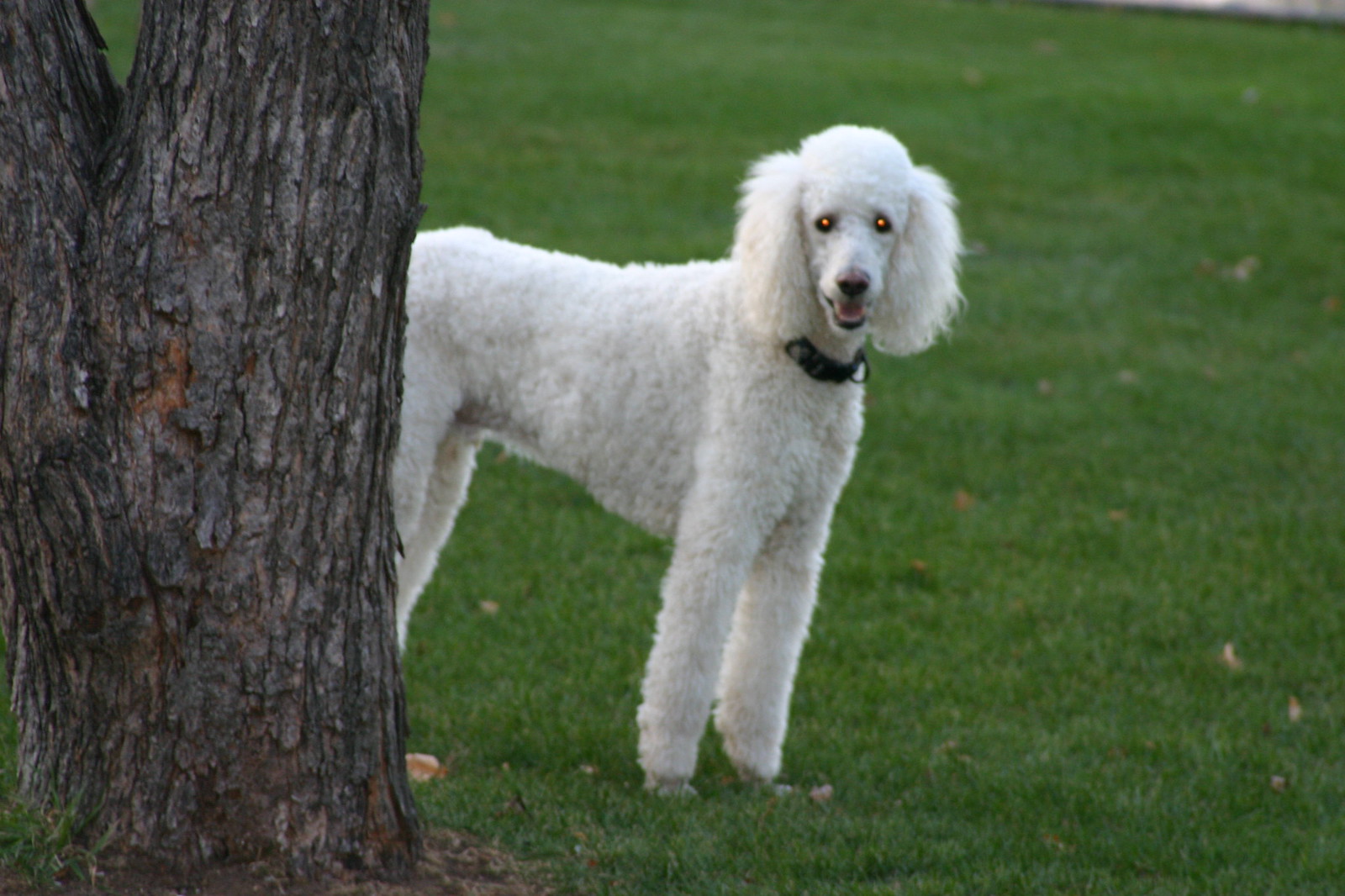A poodle stands proudly on a neatly trimmed green lawn, its curly white fur contrasting against the vibrant grass. The dog's long legs and larger body give it an elegant yet sturdy appearance. Floppy ears frame its expressive face, where its slightly open mouth suggests a relaxed and content demeanor. Around its neck, a black collar with a dangling loop adds a touch of simplicity to its otherwise regal look. To the left in the foreground, the base of a large grey and brown tree trunk emerges from a patch of bare dirt, grounding the scene in a natural setting. The lighting creates a striking reflection in the poodle's eyes, casting an orange-red hue that stands out against the likely natural black or brown of its pupils. The dog's gaze is fixed forward, engaging the viewer with a sense of curiosity and warmth.